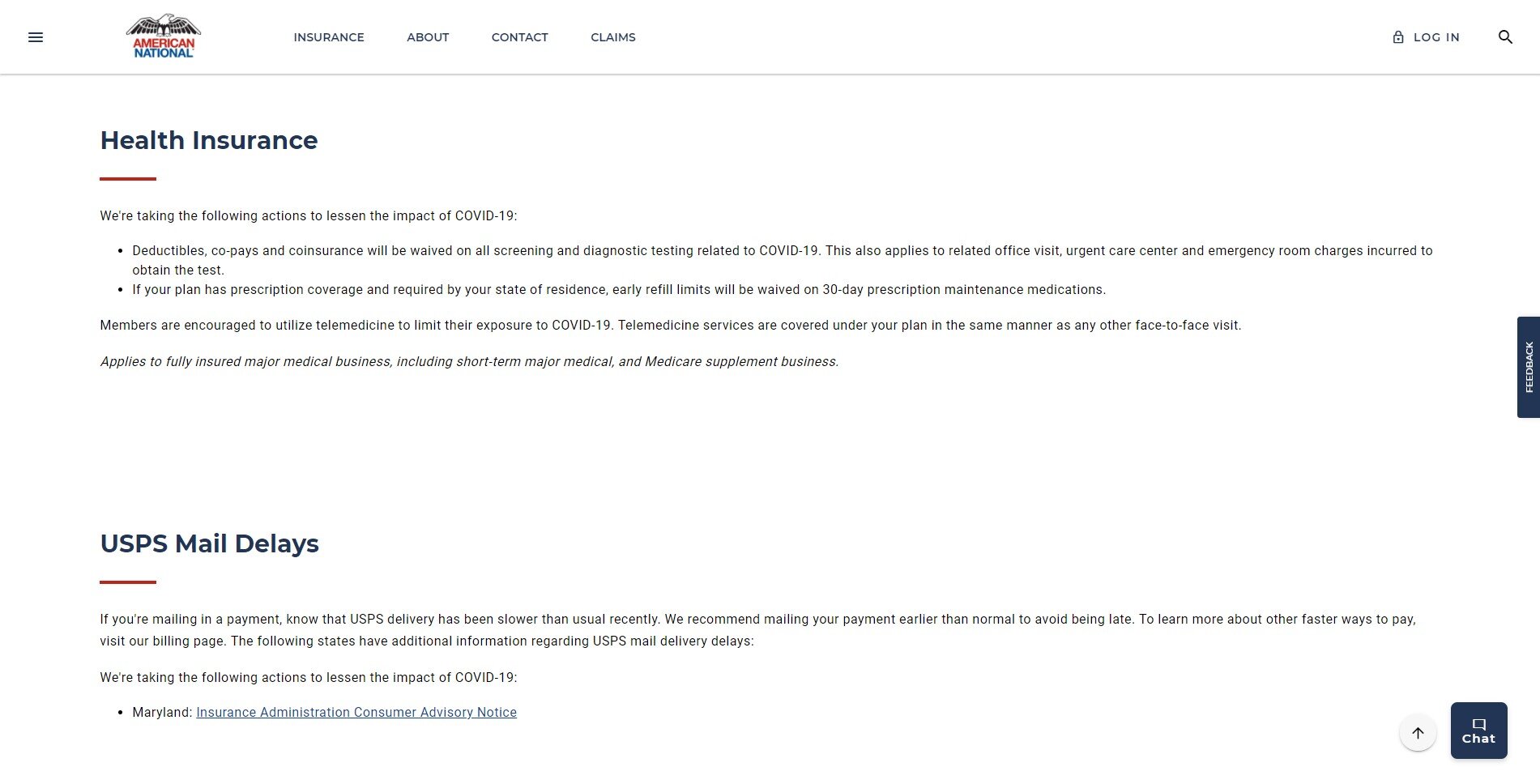This image is a screenshot of the American National Insurance website displayed on a computer browser. 

- **Top Navigation Bar:**
  - In the upper left-hand corner, there are three horizontal lines indicating a drop-down menu.
  - To the right of the menu icon is the American National logo featuring an eagle.
  - Adjacent to the logo are navigation buttons labeled "Insurance," "About," "Contact," and "Claims."
  - On the far right of the navigation bar are a magnifying glass icon (for search) and a login button.

- **Main Content:**
  - The website's background is white.
  - Prominent text near the top reads "Health Insurance" followed by a small red line. 
  - Below this heading, there is a notice regarding COVID-19: "We're taking the following actions to lessen the impact of COVID-19. Deductibles, copays, and coinsurance will be waived on all screening and domestic testing related to COVID-19." However, the text is extremely small and blurry, making it difficult to read further details.
  - Another notice beneath that states "USPS mail delays" followed by a small red line and a brief, unclear block of text.

- **Side and Bottom Elements:**
  - On the far right of the screen, a blue vertical button labeled "Feedback" is visible.
  - At the bottom right-hand corner, there are two buttons: one for initiating a chat, labeled "Chat," and another featuring an upward-pointing arrow for scrolling back to the top.

Overall, the image depicts a detailed layout of the American National Insurance website with a clear focus on the user interface and important informational updates, particularly related to health insurance and COVID-19 measures.